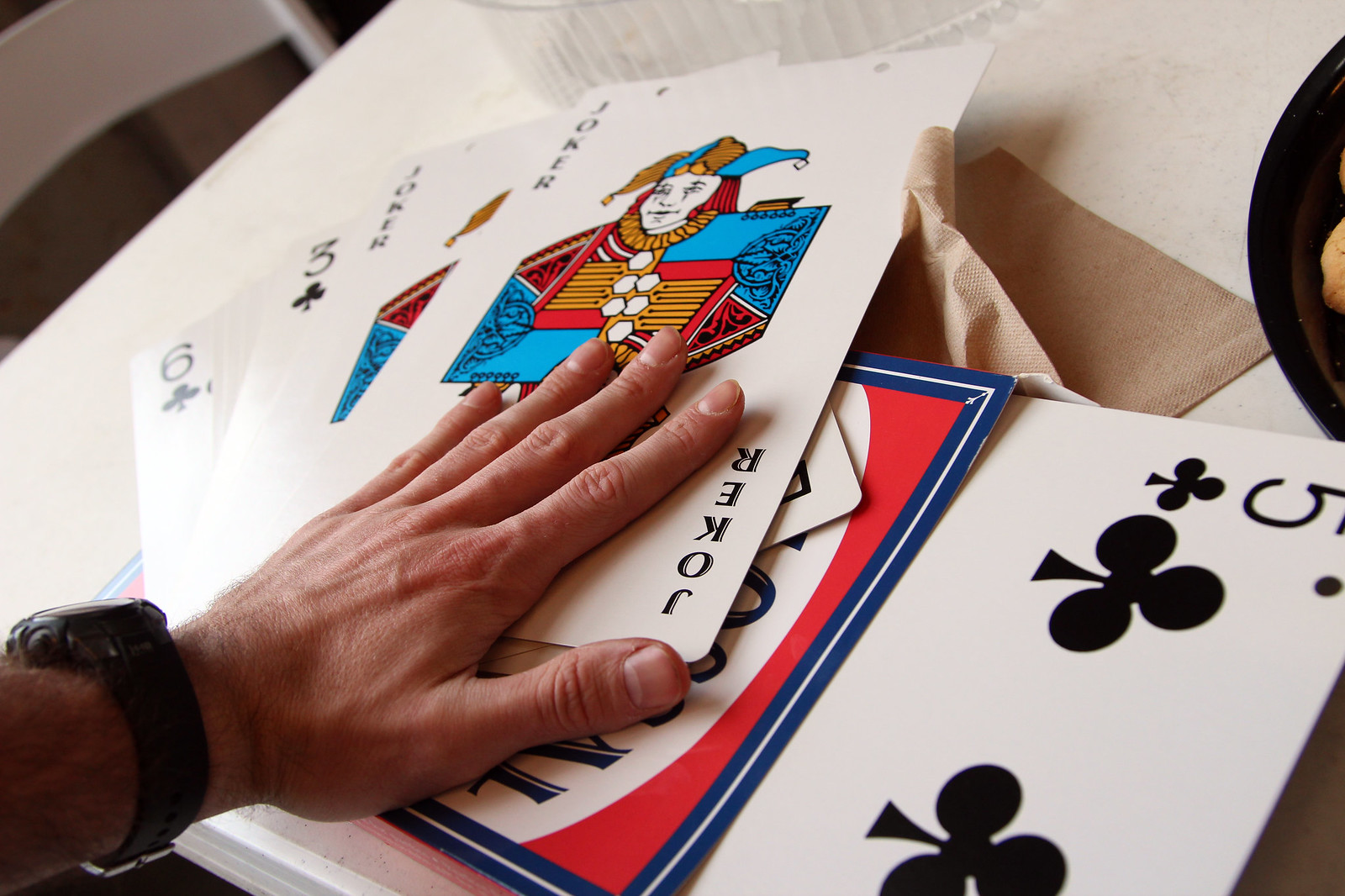This photograph captures a set of jumbo-sized playing cards, significantly larger than standard playing cards, seemingly designed for a stage magic act or as a teaching device. Prominently displayed at the top of the pile is a joker card, distinguishable by two punched holes at the top—presumably for hanging the card on hooks for display on either a horizontal or vertical surface. A person's left hand is positioned over the joker card, suggesting interaction with the cards.

Below the joker card are other oversized cards, including another joker, a three of clubs, a six of clubs, and a five of clubs, all lying on a white table surface. The five of clubs appears to be partially pulled out of a box, likely the original packaging for the jumbo card set, which is placed beneath the cards and the hand. A brown paper towel lies under the pile of cards, adding texture to the scene. Blurred in the background is the indistinct corner of a room, providing context to the setting.